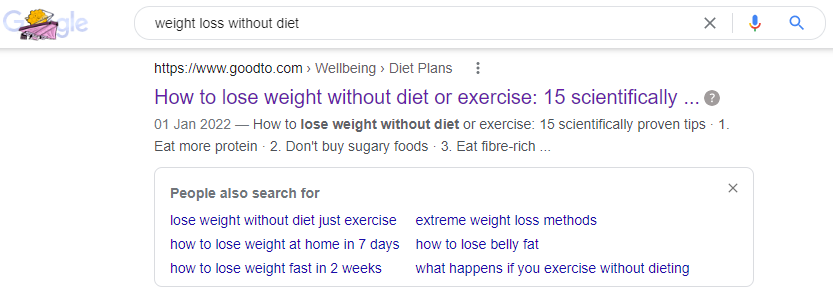This image is a left-to-right horizontal screenshot of a Google search results page, captured from a computer or smart device screen. The background is predominantly white, characteristic of a Google search interface. 

At the top left of the image, the iconic Google logo partially overlaps the search bar, where the query "weight loss without diet" is entered. To the right within the search bar, there are standard interface elements: a gray 'X' for clearing the search input, a microphone icon for voice search, and the magnifying glass icon used to initiate the search.

Beneath the search bar, the web address displayed is "https://www.good2.com," which appears within the usual white screen background. Below this, there are categorized links labeled "Wellbeing" and "Diet Plans," followed by an icon depicting three vertical circles, indicating more options available.

The first search result is partially visible, titled "How to lose weight without diet or exercise, 15 scientifically…" and is cut off by an ellipsis, ending with a question mark. A brief description snippet follows this title. 

Another section labeled "People also search for" appears beneath the first search result, contained within a long rectangular box. This section highlights related search queries in a bluish-purple font, suggesting clickable links. An 'X' is located in the upper right-hand corner of this box to close the suggestion panel.